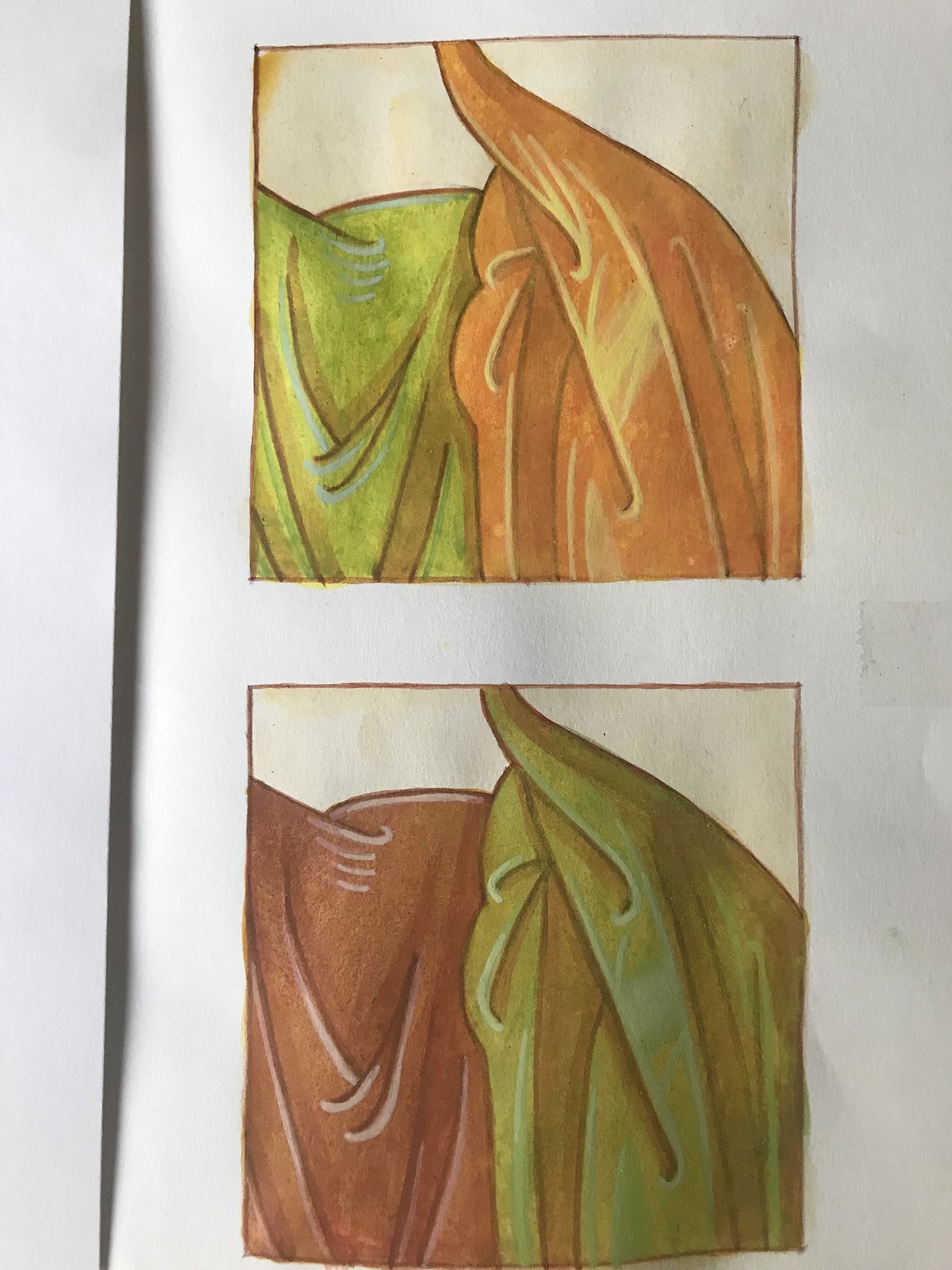The image depicts a page from a book or an artistic panel that is taller than it is wide, featuring two sheets of paper with the top sheet partially obscuring the bottom one, casting a slight shadow. The visible part of the bottom sheet has an off-white color and contains two images, one above the other, each illustrating pieces of fabric-like objects in different colors and arrangements.

The top image showcases side-by-side fabrics with a roughly 10% height gap of white space separating them. On the left is a green draped fabric and on the right is a light red or reddish-brown cloak-like fabric. These images appear to be drawn with colored pencils or a similar medium, giving them a rugged, folded texture.

Below, the second image inversely mirrors the first: the left side features a dark red or maroon fabric, while the right side presents a green moss-like fabric. Both images share a cream or peach-colored background, reinforcing the similarity and contrast between the two sets of fabrics. The detailed textures and folds within the fabrics emphasize a sense of depth and realism in the artwork.